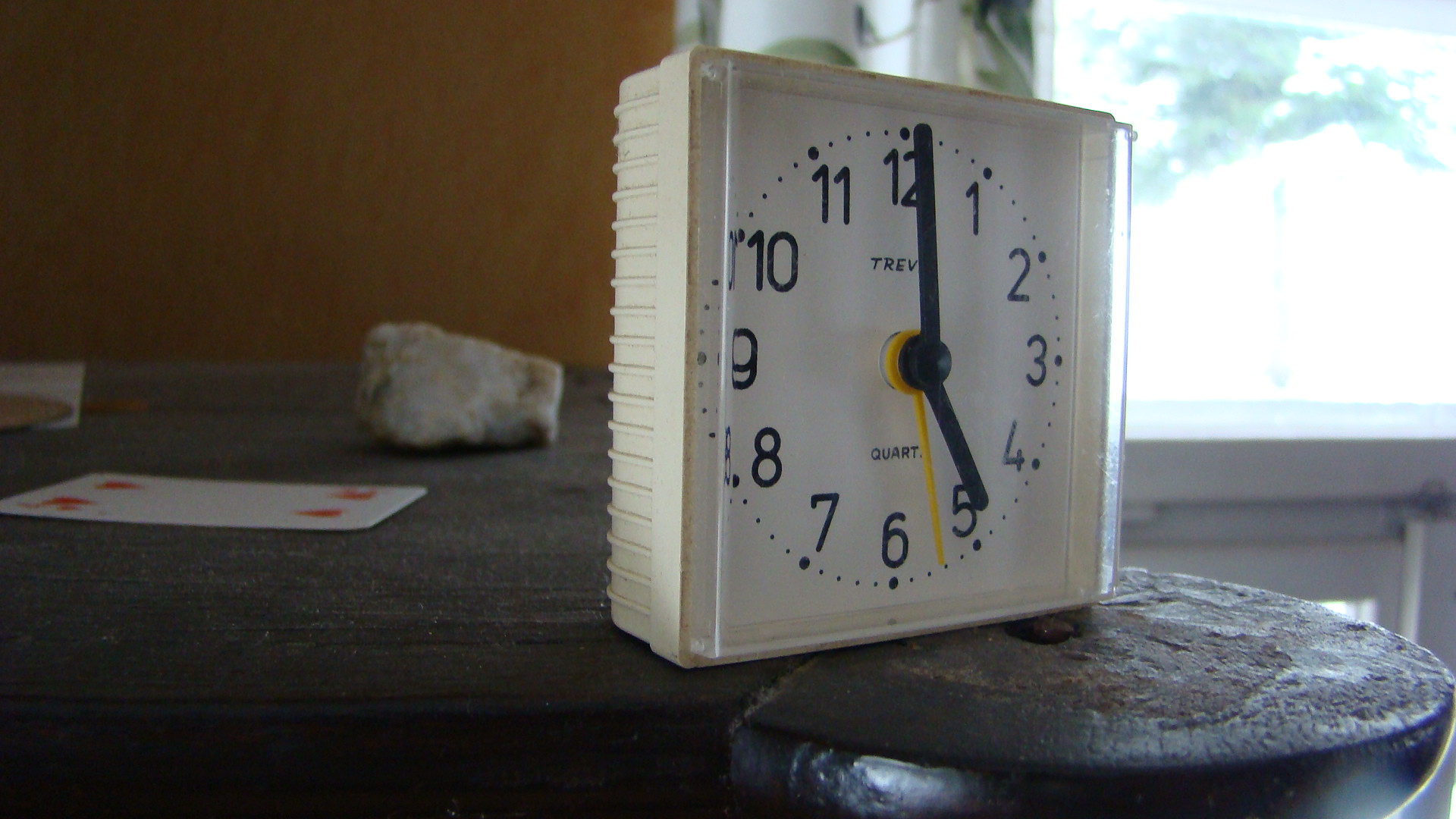This photograph captures a detailed scene featuring a small, square, white plastic alarm clock. The clock, with an acrylic square cover that protrudes slightly, is prominently placed on a roughed-up, black surface laden with white dust and scratch marks. The clock face is also white, adorned with black algebraic numbers from 1 to 12, each hour marked with a black circle. The clock's hands are black, except for the second hand, which is yellow. Notably, the text "TETREV" is inscribed below the 12, and "quartz" is marked above the 6. The clock’s hour hand points at 5, the minute hand at 12, and the yellow second hand at 5:30.

The surface the clock rests on is cluttered with various objects: to its left, there's a playing card, specifically the four of hearts, which is white with red heart symbols. Nearby, there's a rough-surfaced rock, predominantly white with black markings. Toward the back of the surface lies a piece of paper partially covered by an indistinct brown object, maintaining a sense of disarray.

The backdrop includes a dark orange wall and, to the right, a window framed with draping curtains. The window, being open, emits a bright, blown-out light with hints of green foliage visible through it, adding depth and texture to the overall composition. The scene offers a blend of antique and rugged elements, creating a visually rich and narrative tableau.